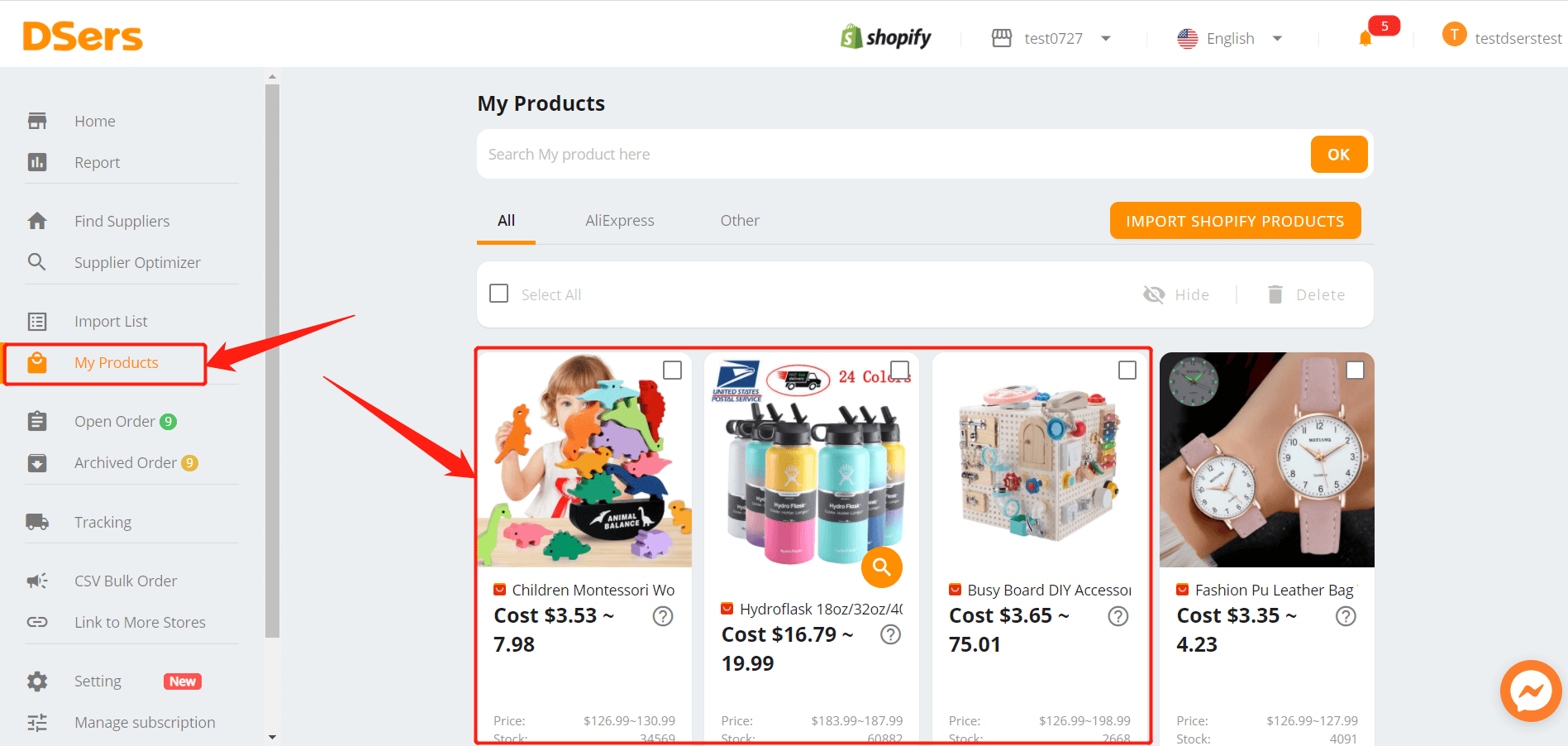The web page features a clean, structured format with a prominent white strip at the top. On the top left corner of this strip, "DSERS" is displayed in an eye-catching orange font. Centrally positioned at the top, the Shopify name is accompanied by its iconic green logo. Adjacent to this, there is a user interface element that includes the user’s username, an image of the American flag, the word "English," and a notification box showing three unread notifications, although these details appear somewhat small and blurry.

Below the white strip, the majority of the page is filled with a large gray box. At the top of this section, the heading "My Products" is prominently displayed. Beneath this heading, there is a search bar accompanied by an orange button labeled "OK." Below the search bar, categories including "All," "AliExpress," and "Other" are listed, with an orange-highlighted box labeled "Import Shopify Products" being particularly noticeable.

In the main product listing area, various items, including a product referred to as "Children's something," are displayed. The price of this item ranges from $3.53 to $7.98. To the right, there are images of water bottles priced between $16.79 and $19.99. The layout is clearly designed to facilitate easy navigation and efficient management of products.